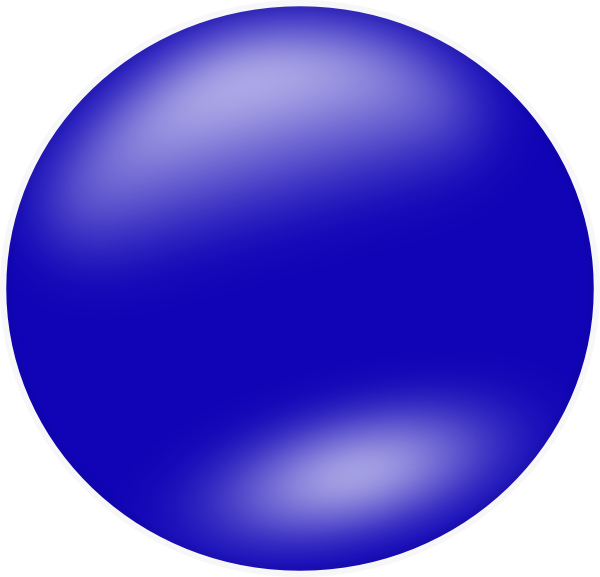The image features an extremely minimalist design with a solid blue background. Centered prominently within the frame is a blue sphere, slightly shaded to give it a three-dimensional appearance. The shading varies, being more pronounced at the top left and bottom right of the sphere, with subtle yellow highlights near these regions. This careful gradation in color adds a gentle depth to the sphere against the plain background. There are no other elements or distractions in the image, ensuring that the focus remains entirely on the blue sphere.